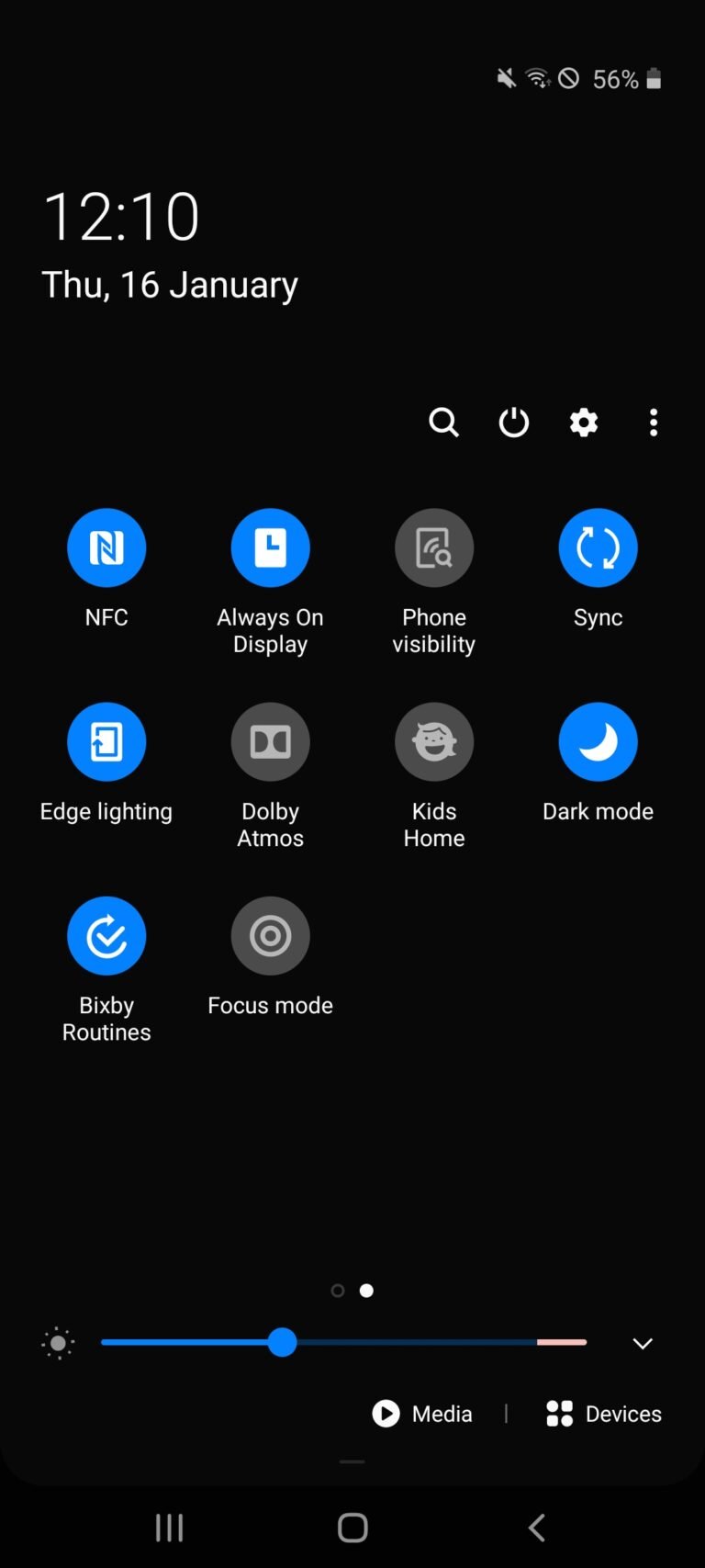In this image, the cell phone screen is being reviewed, specifically in dark mode, featuring a black background. The screen displays that the battery life is at 56% and the current time is 12:10, although it does not specify whether it is AM or PM. The date is shown as Thursday, January 16th. 

Prominently, blue buttons are displayed for adjusting various settings. These settings include:

1. NFC (Near Field Communication)
2. Always On Display, which can be selected to show the date and time continuously
3. Phone Visibility
4. Sync, for synchronizing the phone
5. Edge Lighting
6. Dolby Atmos
7. Kids Home
8. Dark Mode
9. Bixby Routines
10. Focus Mode

Below these buttons is a horizontal line indicating a swipe control that allows switching between light mode and dark mode. Further down, there is a media button and an option to view connected devices, which likely leads to the phone’s app menu.